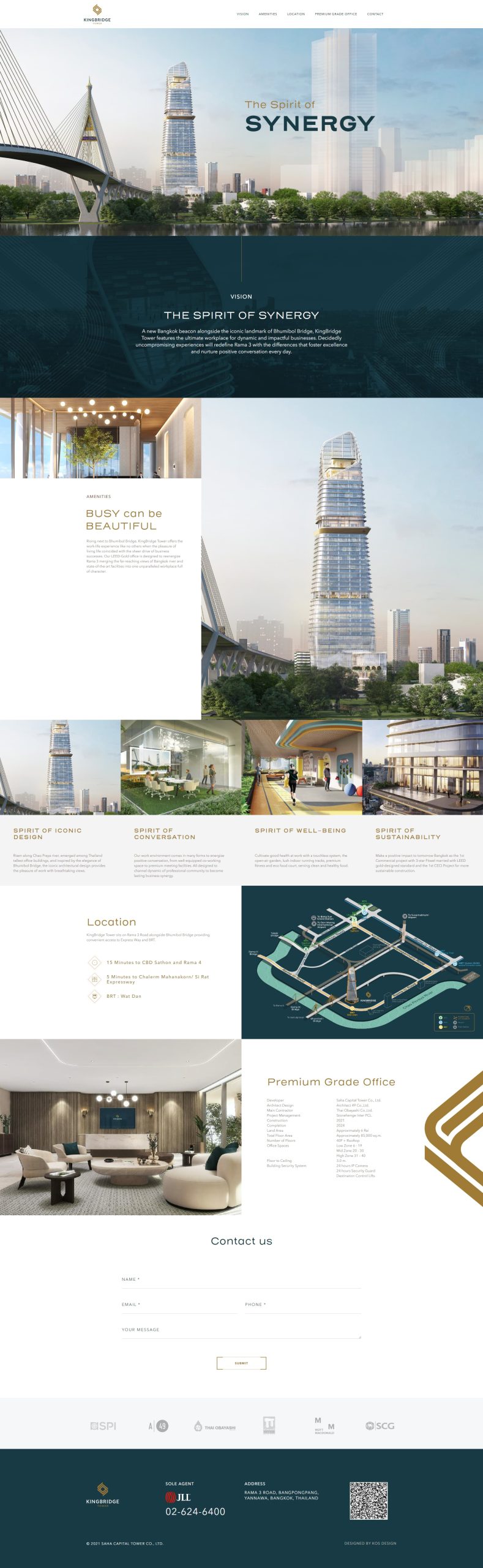Here's the cleaned-up and detailed descriptive caption:

---

The screenshot captures the homepage of a website with a minimalist design. The white header is prominently topped by an elegant gold logo on the top left, which resembles a diamond with radially extending arms. Directly beneath the logo, the name "KINGBRIDGE" appears in bold, all-caps black text, with a line of smaller, blurred gold text underneath it. Spanning the header to the right, ample negative space precedes a navigation menu, featuring all-caps dark gray text that lists: VISION, AMENITIES, LOCATIONS, PREMIUM GRADE OFFICE, and CONTACT.

Below the header, an architectural rendering of a cityscape dominates the image. On the left, a tall suspension bridge boasts numerous cables descending from triangular-shaped towers. Adjacent to the bridge stands a sleek, segmented glass skyscraper, comprising three distinct sections. Further to the right, a translucent view of several skyscrapers forms a row, featuring an exceptionally tall central building. This backdrop is set against a light blue sky dotted with gray clouds. A river flows across the bottom of the image, framed by a grassy lawn shaded by trees.

Positioned atop the central translucent skyscraper, gold text declares, "THE SPIRIT OF," followed by "SYNERGY" in all-caps dark blue text. Below, another photograph showcases the pinnacle of an office tower, shrouded in a darkened, blue-toned filter. At the center of this image, large white text reads: "VISION, THE SPIRIT OF, SYNERGY."

---

This enhanced caption provides a vivid and precise description of the elements depicted in the screenshot, highlighting key features and the overall layout.